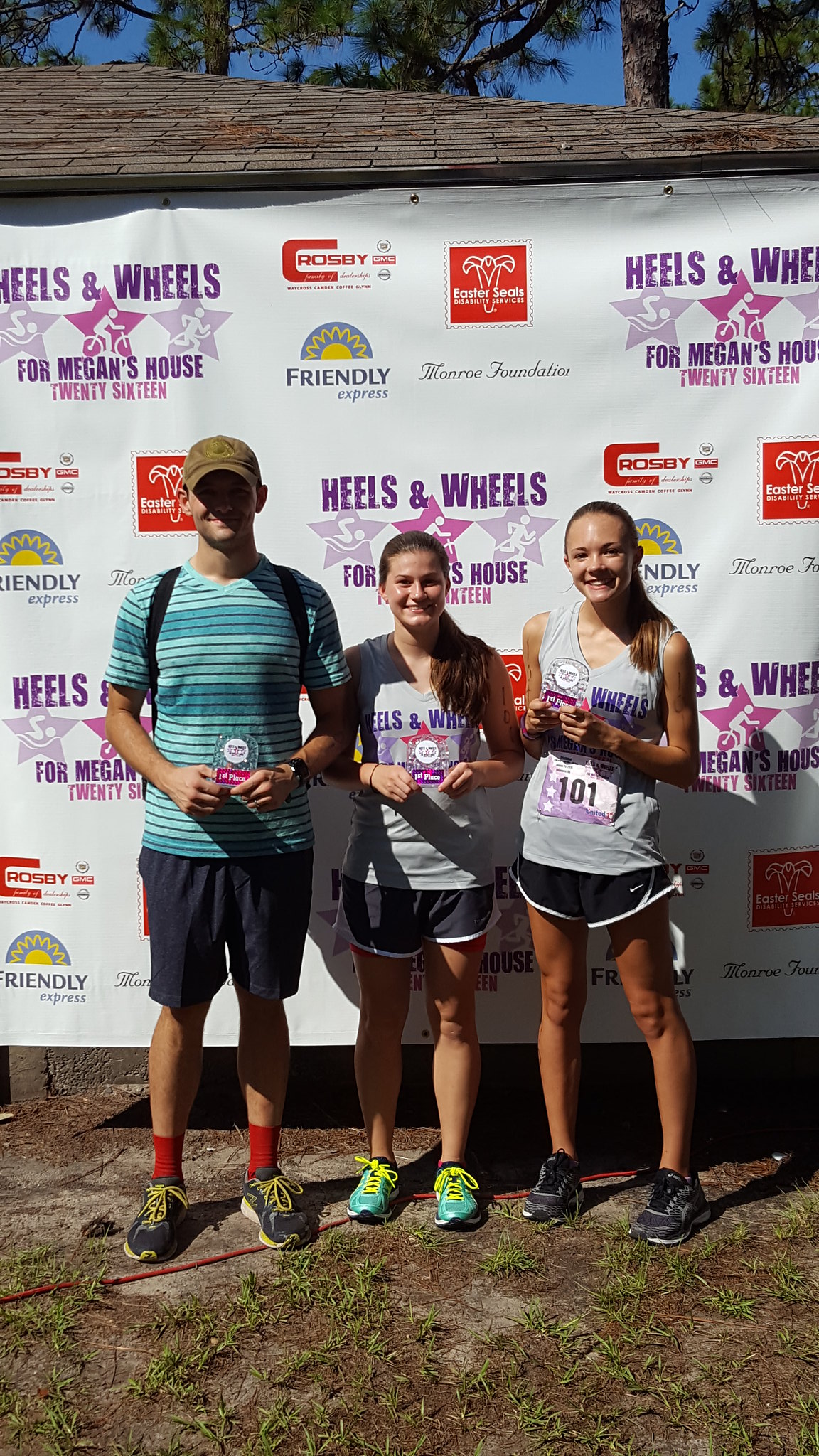The photograph, measuring 4 inches wide by 7 inches tall, captures three participants standing outside at the Heels and Wheels marathon event for Megan's House 2016. They are posing in front of a banner featuring several sponsor logos, including Crosby, Easter Seals, Monroe Foundation, and Friendly Express. The participants, two females and one male, are dressed in casual athletic attire. The female on the left is wearing a gray tank top, black shorts, and black shoes, while holding an award. The female on the right, sporting a black and gray shirt, black shorts, and green tennis shoes with yellow laces, also has an award and is wearing a number tag with '101' on it. The male on the left, who contrasts with a two-tone turquoise t-shirt, a brown baseball hat, dark shorts, red socks, and black shoes, carries a backpack and holds a star-shaped trophy. They are all smiling and standing on a slightly grassy, mostly dirt-covered area, with the backdrop showing trees and the sponsor banner affixed to a small wooden structure.